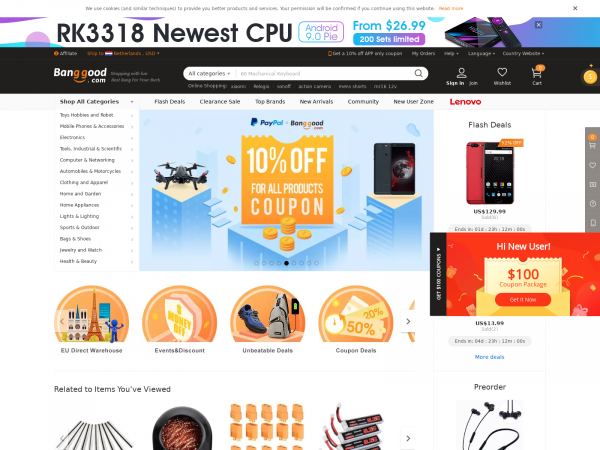The image displays a webpage predominantly featuring a marketing banner at the top with a white background adorned with purple and blue graphics, including circles and lines. The banner promotes the "RK3318 Newest CPU Android 9.0 Pie," stating "From $26.99, 200 sets available, limited time offer."

Below the banner, the page transitions to a black background with the logo "Banggood.com" prominently situated at the top. Adjacent to the logo is a search bar labeled "All Categories," currently displaying the term "mechanical keyboard," with a magnifying glass icon on the right end of the bar.

Continuing along the header, there are options to "Sign In," access the "Wish List" represented by a heart icon, and view the shopping cart.

A navigation menu is located just below, labeled "Shop by Category," though some of the text is difficult to discern. To the right, a blue background features an advertisement with illustrations of buildings, a drone, and a cell phone, alongside the text "PayPal Banggood.com 10% off for all products coupon," accompanied by a stack of coins.

Further down, there are circular icons labeled "EU Direct Warehouse," "Events and Discounts," "Unbeatable Deals," and "Coupon Deals." Below this section, a note indicates items "Related to items you viewed," displaying four different products.

On the right, another section highlights "Lenovo Flash Deals," showcasing a cell phone, alongside a promotional message for new users offering a "$100 coupon package." Additionally, it includes a highlighted "Pre-order" option for earbuds.